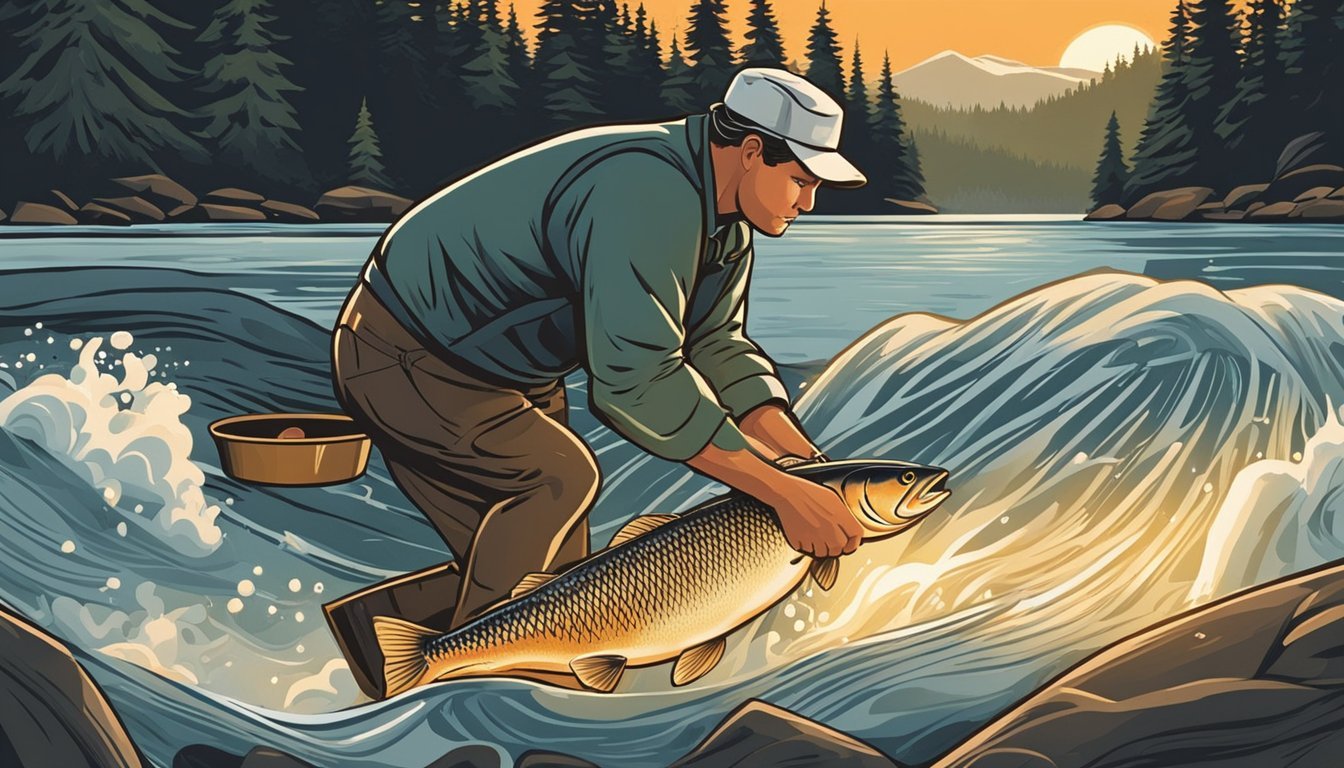The illustration depicts a middle-aged man standing in the midst of a rushing river, gripping a large salmon by its gills. The man, dressed in a long-sleeved blue shirt, long grey pants, and waders, wears a white ball cap on his head and leans slightly forward to manage the impressive catch. Behind him, a gray tin or bowl floats on the water. The background reveals a tranquil expanse of water leading to large grey rocks, tall dark green pine trees, and a dramatic landscape featuring hills clad in dense pine foliage. In the far distance, a majestic snow-capped mountain rises against an orange-hued sky, suggesting the sun is setting. The overall scene has a somewhat stylistic, retro vibe, emphasizing the beauty of the outdoors and the man's successful fishing endeavor.